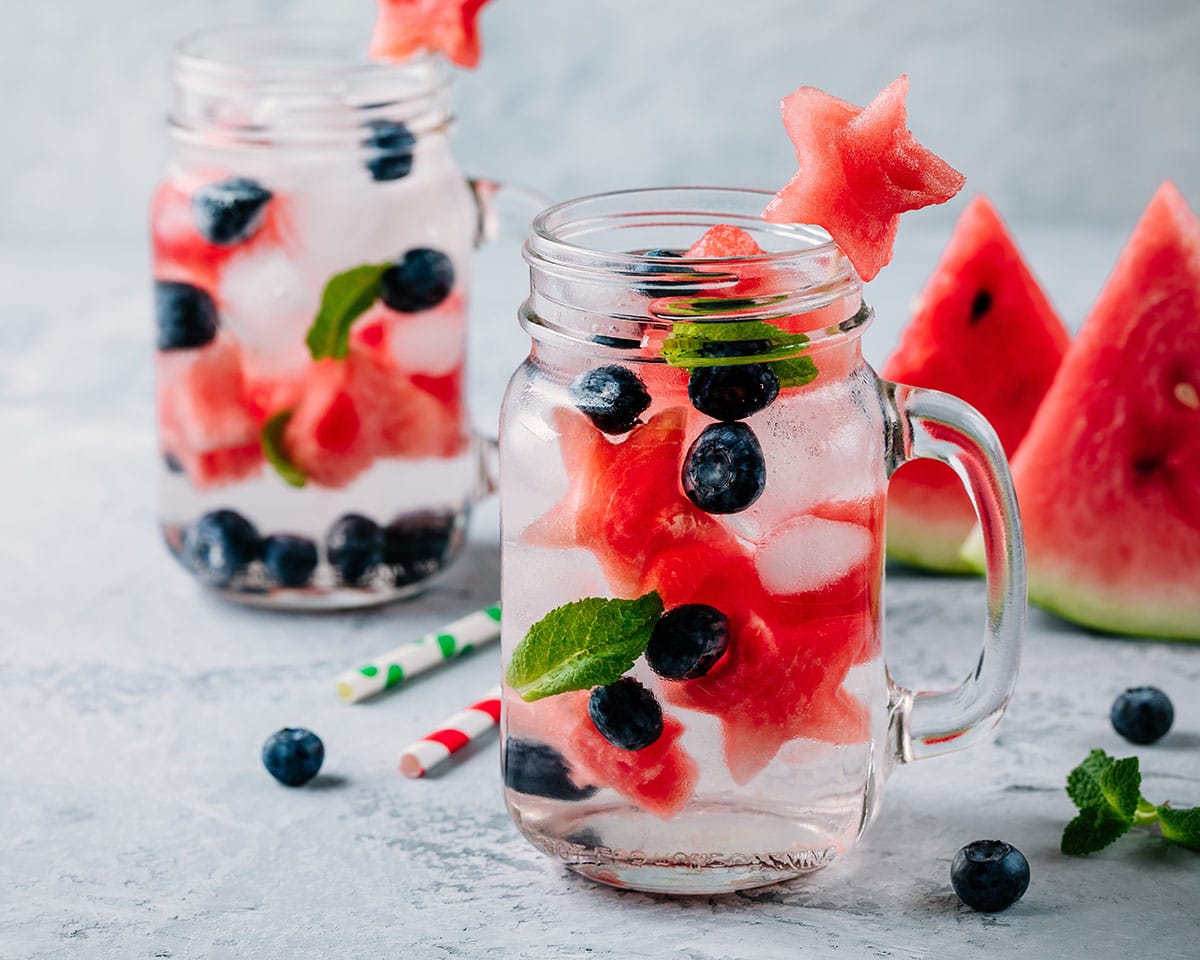This photograph captures a vibrant and refreshing display of two clear mason jar mugs filled to the brim with a refreshing water-based drink, perfectly garnished with summer fruits and mint. Each jar, adorned with a star-shaped watermelon slice perched on the rim, is filled with ice cubes, floating blueberries, and fresh mint leaves. The jars rest on a grey background, creating a contrasting canvas that highlights the bright pink of the watermelon and the dark blue of the berries. In the background, two large slices of watermelon add an extra pop of color, while scattered berries and two straws—a red and white striped one and a white one with green polka dots—complete the lively scene.